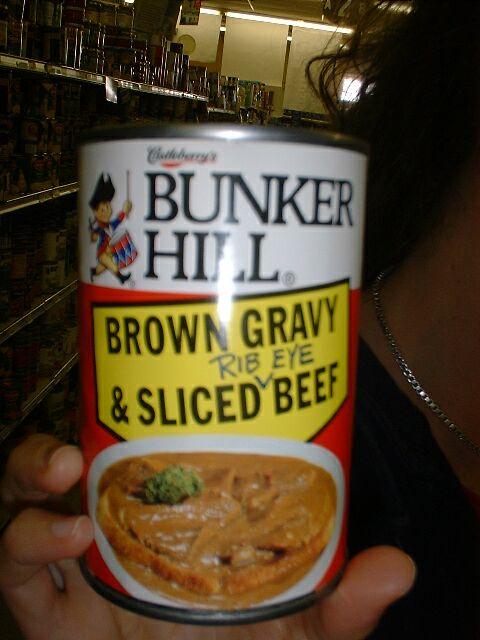The photograph showcases a close-up view of a person with dark brown, curly hair and light-colored skin, wearing a chunky silver-tone chain necklace and a black shirt. Her face is out of the frame, but her neck and outstretched hand are visible holding a cylindrical silver-tone food can. This can features a white, red, and yellow label with black text that reads "Bunker Hill." Adjacent to this text is a small, vintage-style cartoon logo of a drummer boy. Prominently displayed in the center of the label is a yellow flag-shaped tag with black text that reads "Brown Gravy and Sliced Ribeye Beef." Below this description, there is a photorealistic image of a white ceramic bowl filled with the product, depicting the brown gravy and sliced ribeye beef. In the far background, several shelves stocked with canned goods indicate that the setting is likely a retail shop or grocery store. The image's focal point remains on the Bunker Hill can and the surrounding details of its label and contents.